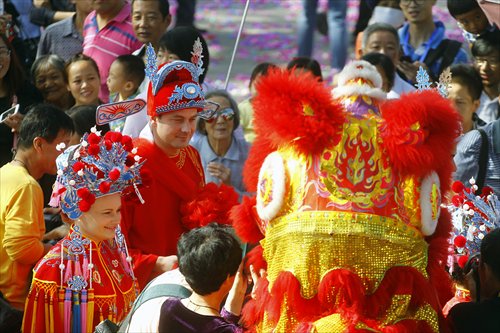In this vibrant outdoor daylight celebration of the Chinese New Year, the bustling street is filled with people, many wearing traditional and festive costumes. Central to the scene is a large, colorful dragon costume adorned with red fluffy ears, golden accents, and red ruffles, moving down the street. Behind the dragon, which features striking white-eyed golden irises and a prominent gold flame on its forehead, are flower petals and confetti scattered across the pavement, hinting at ongoing festivities.

A smiling woman with pale skin and wearing an elaborate traditional dress stands at the forefront. Her red robe is complemented by a blue and red headdress decorated with pom-poms, which dangle over her body. Beside her is a taller man, also smiling, dressed in a similarly festive red costume with a blue-trimmed hat reminiscent of an emperor’s headdress. They appear to be guiding the dragon, which is facing towards the camera with its vibrant red and gold head.

In the background, a diverse crowd, including both Asian and non-Asian individuals, watches the parade with amusement, some wearing costumes themselves. The atmosphere is alive with cultural richness, marked by the dragon and the traditional New Year attire, symbolizing health, wealth, and prosperity.